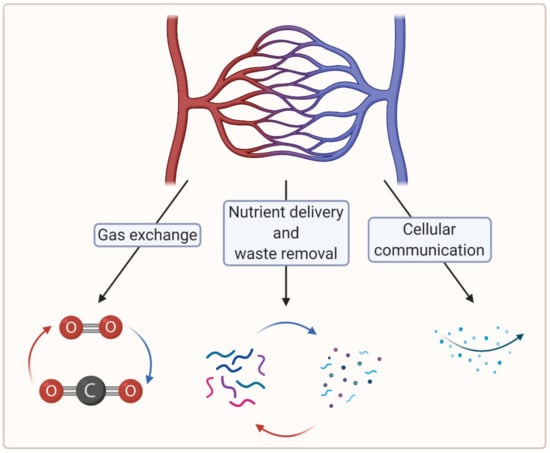This detailed infographic appears to be from a biology or chemistry textbook, illustrating a cell function diagram against a cream-colored background. At the top, there's a representation of interconnected red and blue structures, indicative of a blood or vein system. The central focus of the diagram is divided into three sections, each explaining a different biological process through arrows and symbols:
1. **Gas Exchange:** This section features arrows and cycles describing the process of gas exchange, highlighted with red and blue squiggly lines and symbols such as "O=O" and "CO=O".
2. **Nutrient Delivery and Waste Removal:** Displayed through downward arrows and loops, this part illustrates the continuous cycle of delivering nutrients and removing waste.
3. **Cellular Communication:** Represented by blue dots and curved arrows, this panel shows the process of cells communicating with each other.

Overall, the infographic uses clear, color-coded visual elements to depict the dynamic processes of gas exchange, nutrient delivery, waste removal, and cellular communication within a biological system.